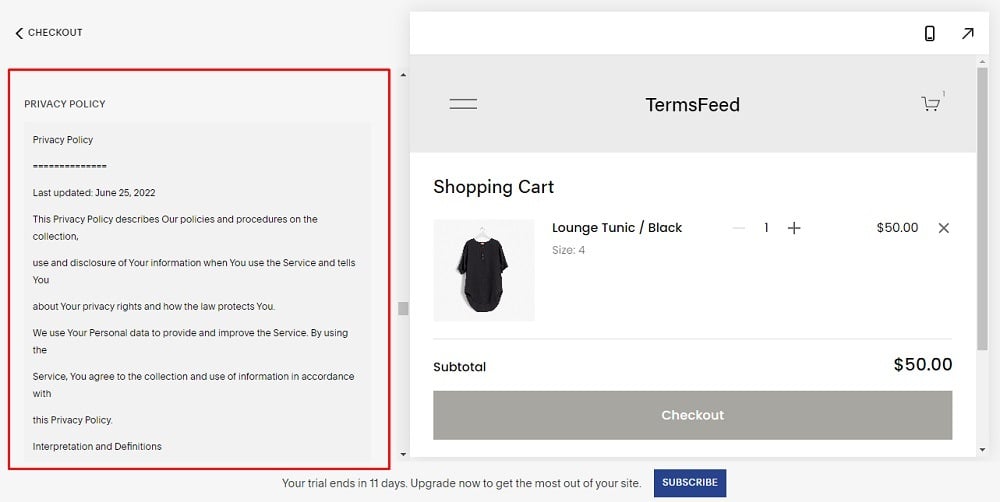A clear smartphone screen displaying a privacy policy statement is visible. The policy, last updated on June 25, 2020, outlines the practices and procedures for collecting, using, and disclosing user information, emphasizing users' privacy rights and how they are protected under the law. It mentions that personal data is used to provide and enhance the service, with usage signifying agreement to the policy.

Below the policy text, there are sections and icons representing data, currency, and a shopping cart. The page includes product details such as a "Lounge Tunic/Pack," available in size four, priced at $50. To the right, control buttons for adjusting the quantity and a gray 'X' for removing items are visible. A subtotal section shows the amount as $50. The checkout button is highlighted within a gray rectangle.

Additionally, a prompt informs the user that their trial will end in 11 days, suggesting an upgrade to maximize site benefits. A blue rectangle with a check box at the bottom of the page states "Subscribe."